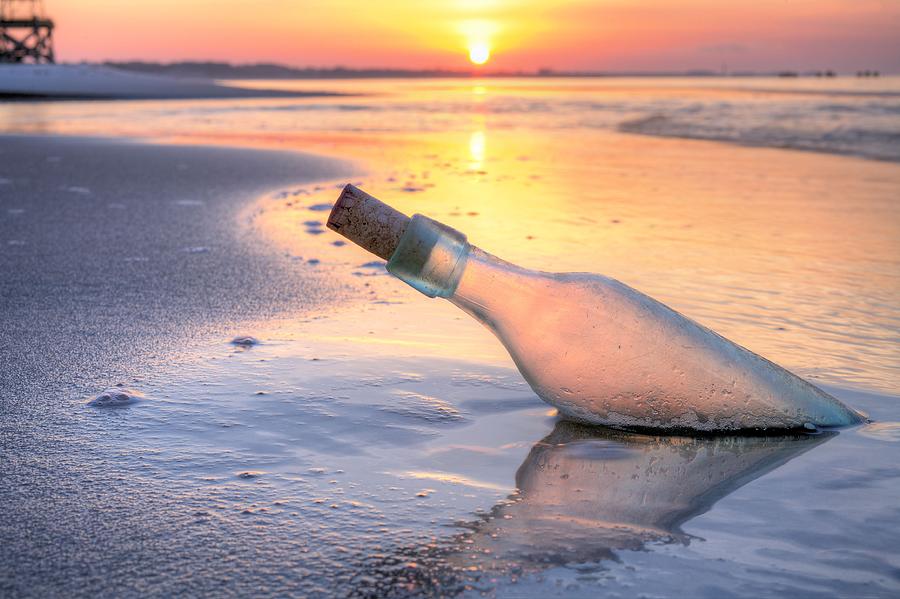The image captures a serene beach scene during either sunrise or sunset, with the golden glow of the sun illuminating the horizon. In the foreground, a clear glass bottle with a brown cork is half-buried in the muddy, gray sand, which reflects the light with a subtle shimmer. The bottle, resembling a classic 'message in a bottle,' adds an element of mystery and nostalgia. Gentle waves bubble and roll onto the beach, and you can see a faint structure, possibly a pier, in the distance on the left. The overall scene is reminiscent of a pastel watercolor painting, adding to the tranquil beauty of the setting.